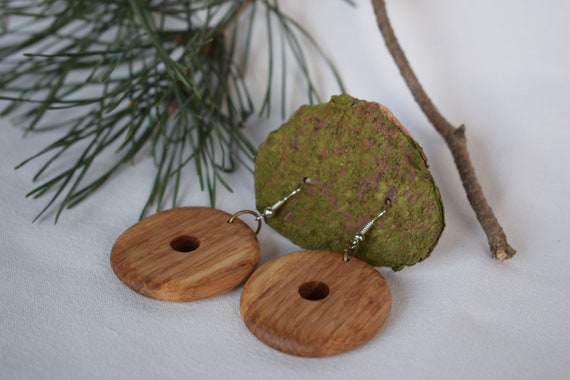This detailed color photograph features a pair of light brown, polished wooden hoop earrings displayed against a textured white background. The earrings are comprised of large, smooth wooden discs with smaller circular cutouts at their centers, suggesting a minimalist design. Each earring is connected by silver metal pins to a green, moss-covered earth-like object, adding a natural, earthy touch to the presentation. Near the earrings, a small twig adorned with conifer leaves enhances the organic aesthetic. The overall composition, with its interplay of wood, metal, and moss, highlights the rustic elegance of the earrings in a serene, white setting.